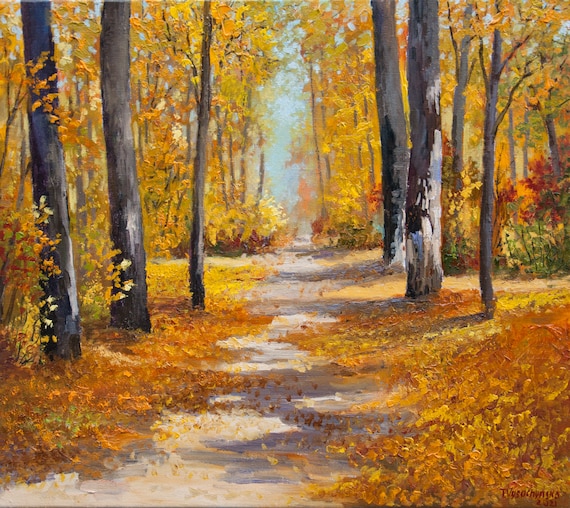This square canvas painting captures the serene beauty of an autumn forest. A dirt trail extends from the bottom center, leading you deep into the scene where it meets a blue-gray sky visible through a canopy of trees. The path is scattered with autumn leaves in shades of orange and yellow, blending seamlessly with the forest floor on both sides, which is thickly carpeted in the same fall hues. Tree trunks, varying from thin to medium thickness, line the trail. These trunks appear in shades of brown, black, and gray, accented with white highlights, creating a striking contrast with the golden foliage. The leaves on the trees mirror the vibrant yellows, oranges, and deep reds of the fallen ones. The artist's name can be seen printed in the lower right corner, though it is hard to distinguish against the similarly colored background. Despite the overall lack of intricate details, the painting vividly conveys the tranquil and immersive atmosphere of an autumn woodland path.